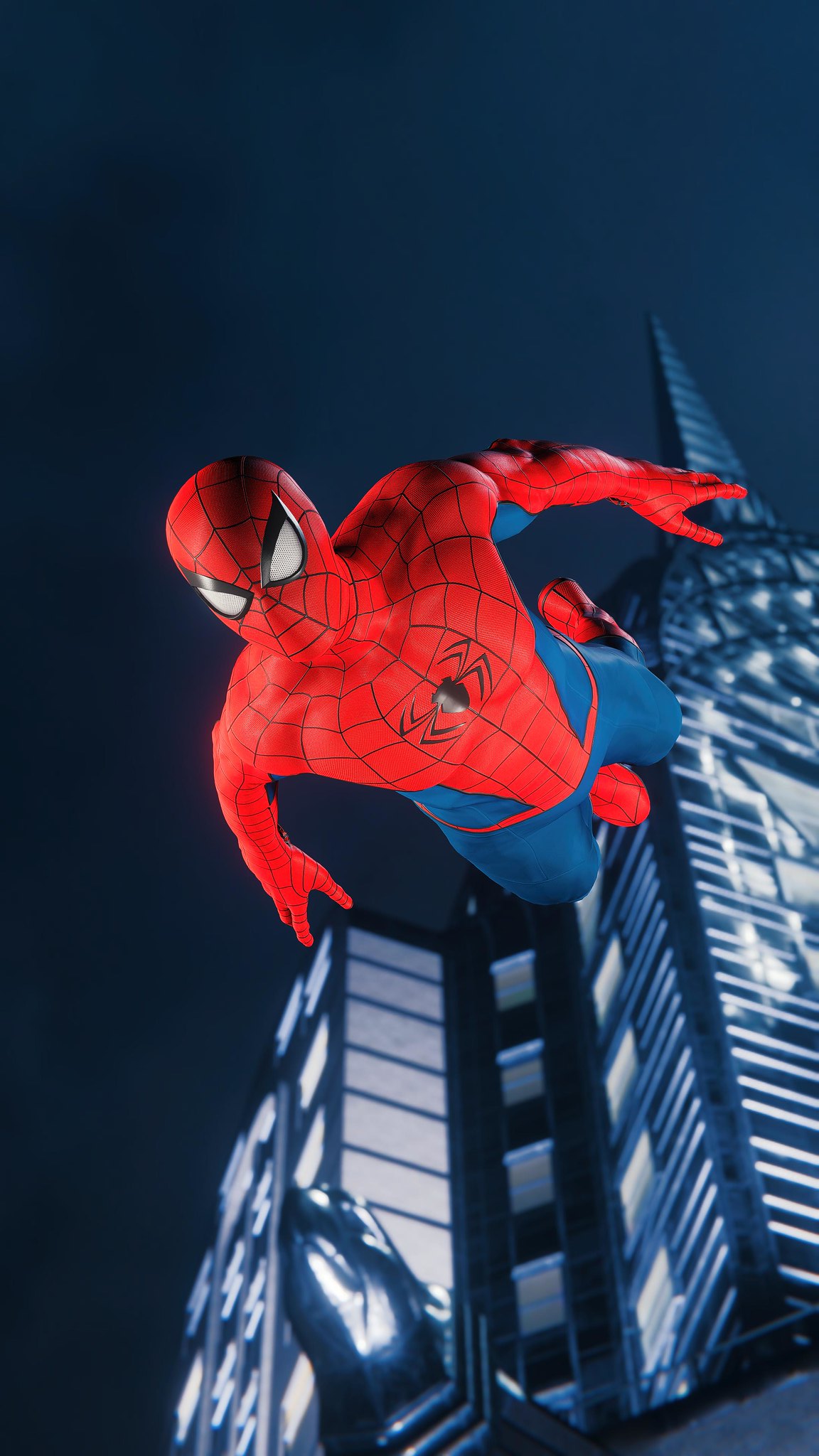This digital artwork depicts Spider-Man mid-action as he descends headfirst toward the ground with a sense of urgency. Behind him, a towering skyscraper with a rounded front and a striking, sharp pyramid-like peak rises dramatically against a dark, ominous sky. Spider-Man, clad in his iconic red suit adorned with a distinctive black spider emblem and detailed with black webbing patterns, appears to be in a dynamic free-fall. His blue pants contrast sharply with his red suit, and additional blue accents around his waist are prominently visible. His arms are extended backward, and his knees are bent, positioning his legs behind him. Notably, the posture reveals the sole of his back foot peeking between his legs, emphasizing his agility and acrobatic prowess. The scene captures the thrilling, high-stakes world Spider-Man navigates.